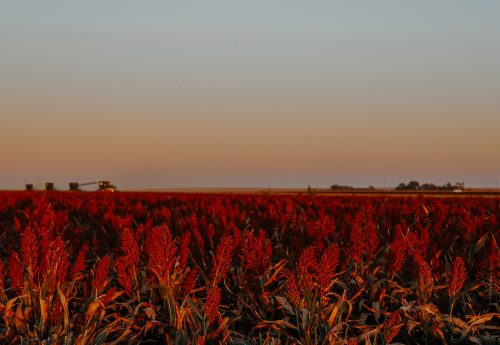The image depicts a vast, outdoor field covered in tall, red, wispy plants with little red flowers at the tips of each stalk, interspersed with green grass at the bottom. The field stretches out beneath a sky that transitions from light blue to gray, fading into hues of yellow and orange, suggesting a sunset scene. On either side of the field, there are white structures resembling houses or farm buildings. In the middle left of the image, several tractors and other farm machinery can be seen, indicating that this is a functional farm. The background includes a line of trees and additional buildings, which are framed by the setting sky. The entire scene captures the serene and industrious atmosphere of a farm at dusk, with its machinery ready for the next day’s work.